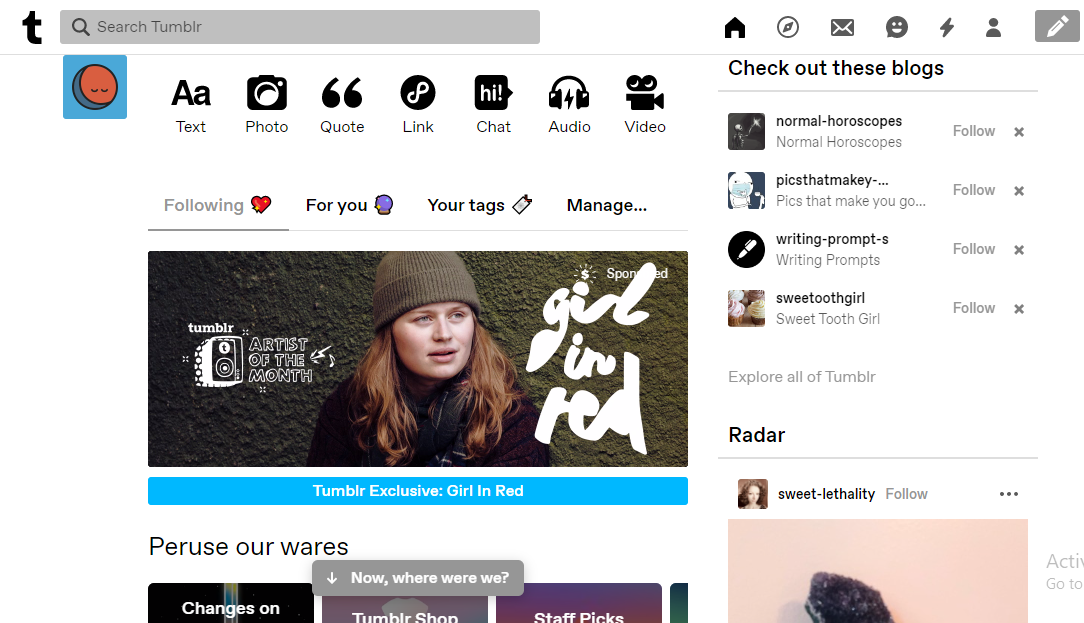A detailed screen capture of a Tumblr webpage reveals its diverse interface and navigation options. At the top of the page, the recognizable Tumblr 'T' logo is visible, accompanied by a search bar labeled "search tumblr." Navigation icons line the top, including Home, Mail, Emoji, Lightning bolt (likely notifications), Account, and Post buttons. Below these options, users can choose from various content types to post, such as Text, Photo, Quotes, Links, Chat, Audio, and Video.

On the right side of the screen, there's a section titled "Check out these blogs," featuring four different blogs that users can follow, along with a hyperlink to "explore all tumblr." Below this section, a widget named "Radar" displays a partially cut-off image linked to the blog "Sweet Lethality," promoting a featured blog post for users to explore.

On the left side, beneath the primary navigation icons, a highlighted Tumblr post showcases "Tumblr Exclusive: Girl in Red." This post includes an image of an artist with red hair and a beanie, labeled with "girl in red" in a funky script, the Tumblr logo, and the designation "Artist of the Month." This content is marked as sponsored. Below this, options for "following," "for you," "your tags," and "manage..." are partially visible for user interaction. Further down, there's an incomplete section titled "Peruse our wares," with cut-off icons hinting at more navigation options not fully displayed in the capture.